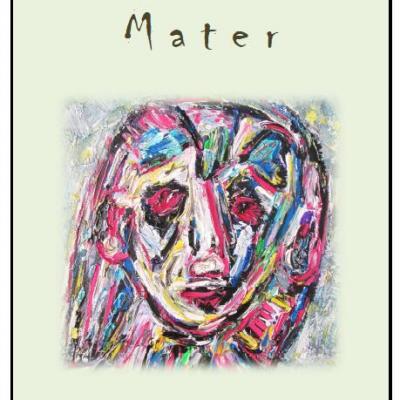The image portrays an abstract, cartoonish face rendered in a riot of colors including blue, pink, white, red, brown, yellow, and green, set against a very light green background. At the top, in darker, slightly fancy lettering, is the word "Mater" written in black ink. This could potentially be interpreted as either an album cover or an advertisement for an art gallery exhibit. The abstract face features distinct but unconventional elements: the eyes have red circles around black irises, the nose is notably long and either deformed or exaggerated, with white on the left side and red on the right. The figure has an outline of U-shaped hair that blends multiple hues, including blue, white, yellow, and green.